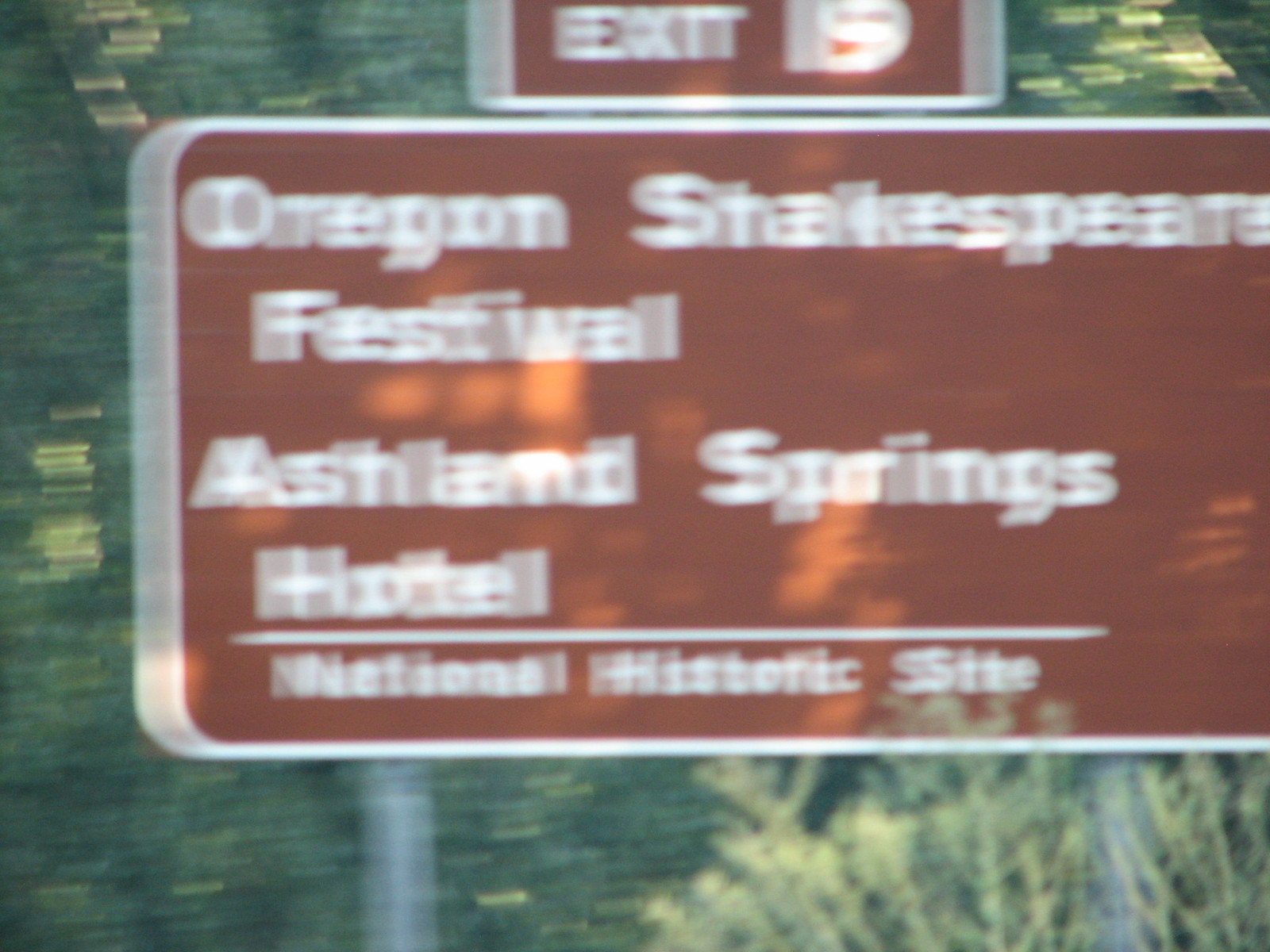This photograph captures a brown highway sign taken from a moving vehicle, evident from the noticeable motion blur. The rectangular sign, with curved edges and a white border, stands against a backdrop of vibrant green foliage including trees and bushes. Despite the blur, the text on the sign is discernible: "Exit 19" at the top, and below it, "Oregon Shakespeare Festival, Ashland Springs Hotel, National Historic Site." The close-up shot emphasizes the sign's directional information while providing a fleeting glimpse of the lush roadside scenery.